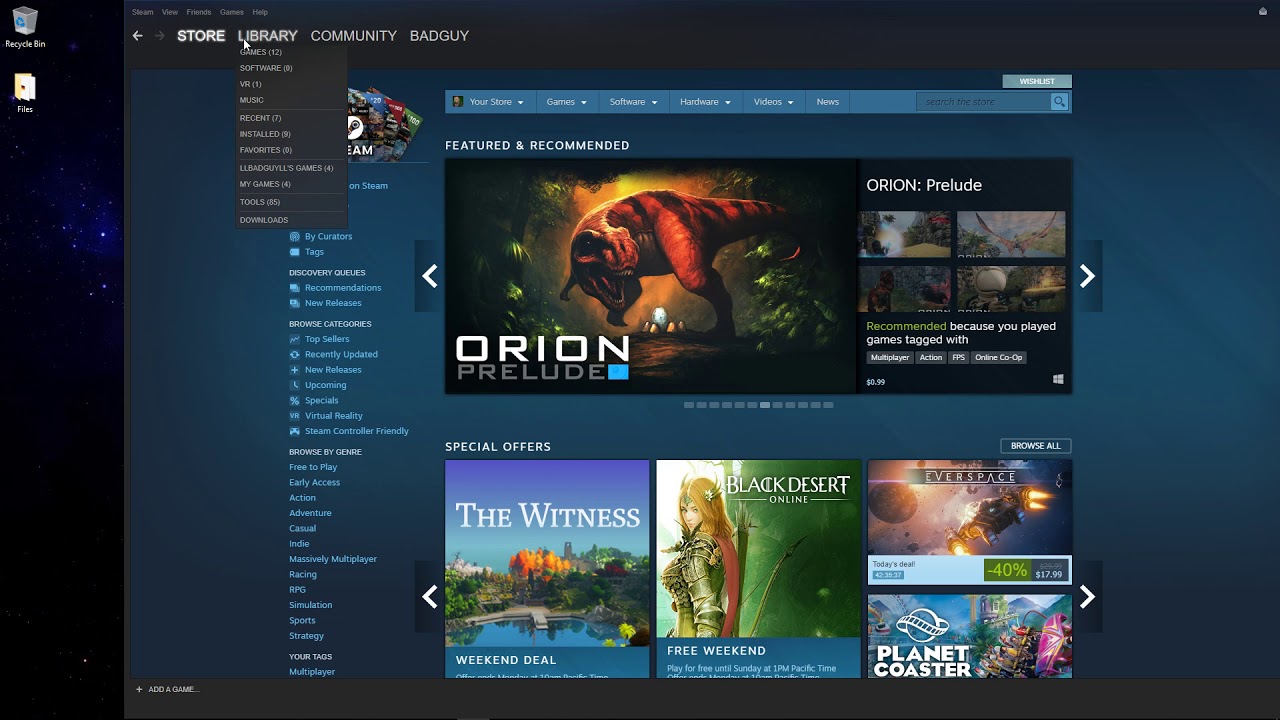The screenshot features the Steam client open on a Windows computer. The Store tab is currently active, showing the featured item "GamePod Orion Prelude," which prominently displays dinosaurs. The user's mouse cursor is hovering over the "Library" section. The Steam user is identified by the username "LLBADGUYLL" and has the display name "BADGUY" (all uppercase, no spaces). This user possesses 12 games in their Library, with one VR title. The user also has 85 codes. Below the featured item, there are special offers listed, including "The Witness," "Black Desert Online" for a Free Weekend, "Everspace," and "Planet Coaster." The screenshot captures a typical view of the Steam Store interface.